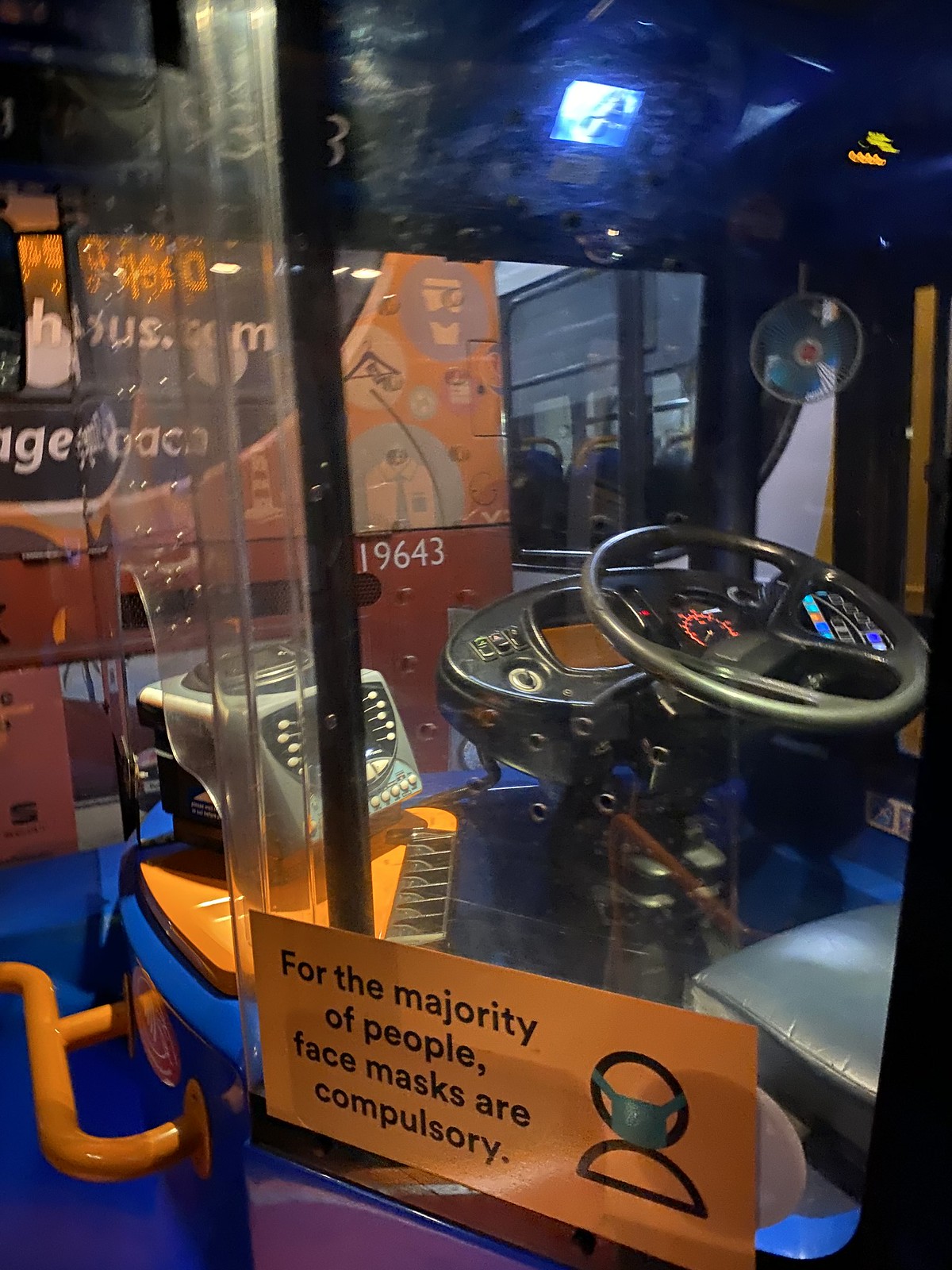The image portrays the driver's seat of a bus, viewed from an external vantage point through a window. It features a black seat positioned up high, suggesting it's a bus driver's cockpit. The black steering wheel and a partially visible dashboard with various buttons are highlighted. An orange sign affixed to a plexiglass divider reads, "For the majority of people, face masks are compulsory," accompanied by a stick figure in a green mask. The scene also includes a transparency into the front windshield, where another city bus is visible, indicating that the bus is parked behind it. The layout includes an orange handlebar for boarding and blue hues within the interior, reinforcing the pandemic context during which the image was likely taken.